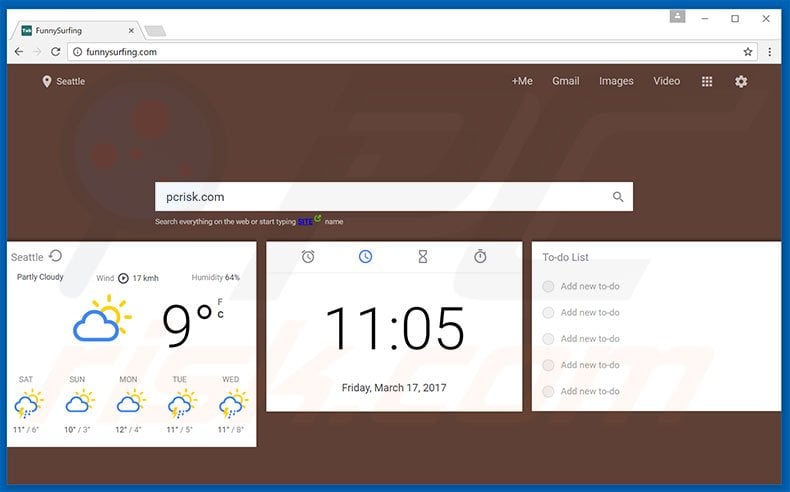A detailed caption for the described image would be:

"A screenshot of a web browser window open to the website 'funnysurfing.com.' The browser displays a single tab in the upper left corner. The background behind the browser is predominantly blue. The web address 'funnysurfing.com' is visible in the address bar. On the website's upper-left section, there is an indication that the location is Seattle. To the right of this location detail, a horizontal menu is visible, featuring options such as 'Menu,' 'Plus,' 'Me,' 'Gmail,' 'Images,' and 'Video.' Further to the right, there is a grid icon made of smaller squares and a gear icon representing settings. Below this navigation bar, there is a centered search bar with 'pcrisk.com' typed into it. Beneath the search bar, three larger boxes are visible, aligned horizontally, displaying information for the weather, the current time, and a to-do list."